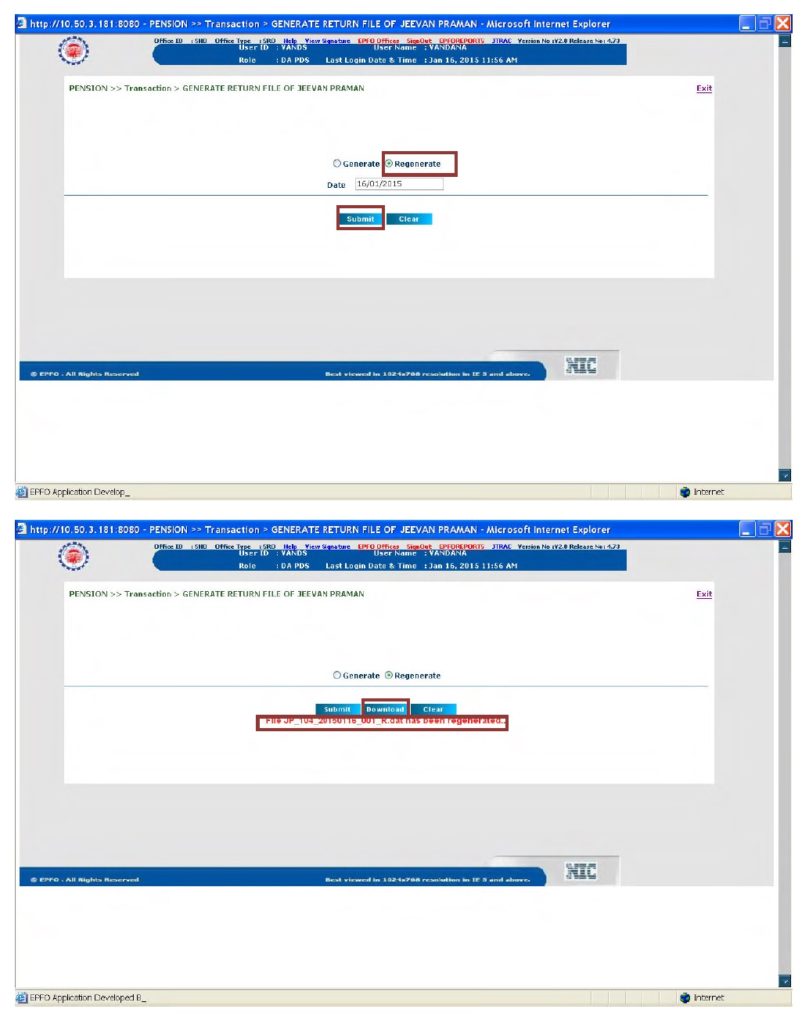The image consists of two vertically stacked screenshots, both displaying the same admin login panel from an Internet Explorer browser window. The panel header features a blue tab at the top-left corner adorned with the Internet Explorer icon, while the top bar contains white text, though it is not legible due to the zoomed-out view.

Below the header, there is a section with several options, which have been obscured by a blue line for privacy or clarity. Beneath that, the main body of the panel shows a large gray box at the top, while the remaining space is blank white. Within this gray box, there are two regions highlighted in red rectangles, indicating areas of significance. One rectangle is positioned at the top-right corner, and another is at the bottom-left around a blue button.

The second screenshot mirrors the first, again focusing on the same panel but with additional annotations. Specifically, there are red text and highlighting around a central option, drawing attention to a blue button in the middle.

Overall, the screenshots illustrate a heavily annotated admin login panel where critical elements are emphasized with red highlights and obscuration marks to direct attention to possibly sensitive or functional components of the user interface.